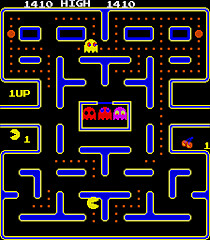This square photograph captures a classic Pac-Man arcade game screen with a detailed black background and a maze made of navy blue T-shapes and rectangles outlined in thin yellow lines. The primary character, Pac-Man, is depicted in bright yellow as he navigates the maze, chomping through numerous small red dots. The objective is to avoid being caught by the animated ghosts, of which there are four distinctly colored ones: red, pink, light purple, and yellow. Specifically, three ghosts—red, pink, and light purple—are seen "locked" in a central white rectangle, often considered the "jail" area, waiting to be released into the maze. Another yellow ghost is already moving around the maze. At the top of the screen, the game displays a score of "1,410 high" and "1,410," highlighting that this is the current and possibly the highest score attained in the game. Additional elements include a cherry on the right side of the screen, which signifies extra points, and a narrow, thin white band at the bottom. The text on the top of the screen provides informative gameplay details, enhancing the overall retro aesthetic of the iconic Pac-Man game.